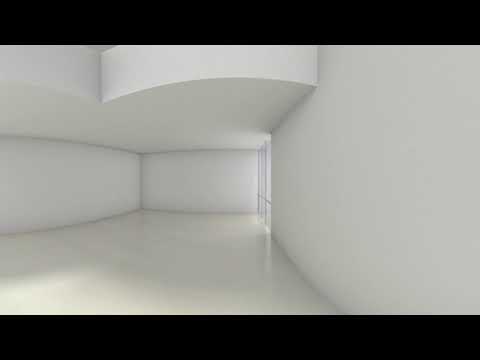The image depicts a spacious, unadorned white room with curved, convex walls that give it a unique and modern feel. The flooring and ceiling are also white, contributing to the room's pristine appearance. Noteworthy is the ceiling's design, featuring areas that appear to be lowered, creating interesting spherical shapes. Positioned towards the center-right of the room is an entryway, seemingly gated, from which light emanates, adding a focal point to the otherwise austere space. The image is framed by relatively thick black borders at the top and bottom. Overall, the room's minimalist design is accentuated by the absence of people and furniture, making its architectural details stand out more prominently. The nature of the image suggests it might be a digital drawing rather than a photograph.